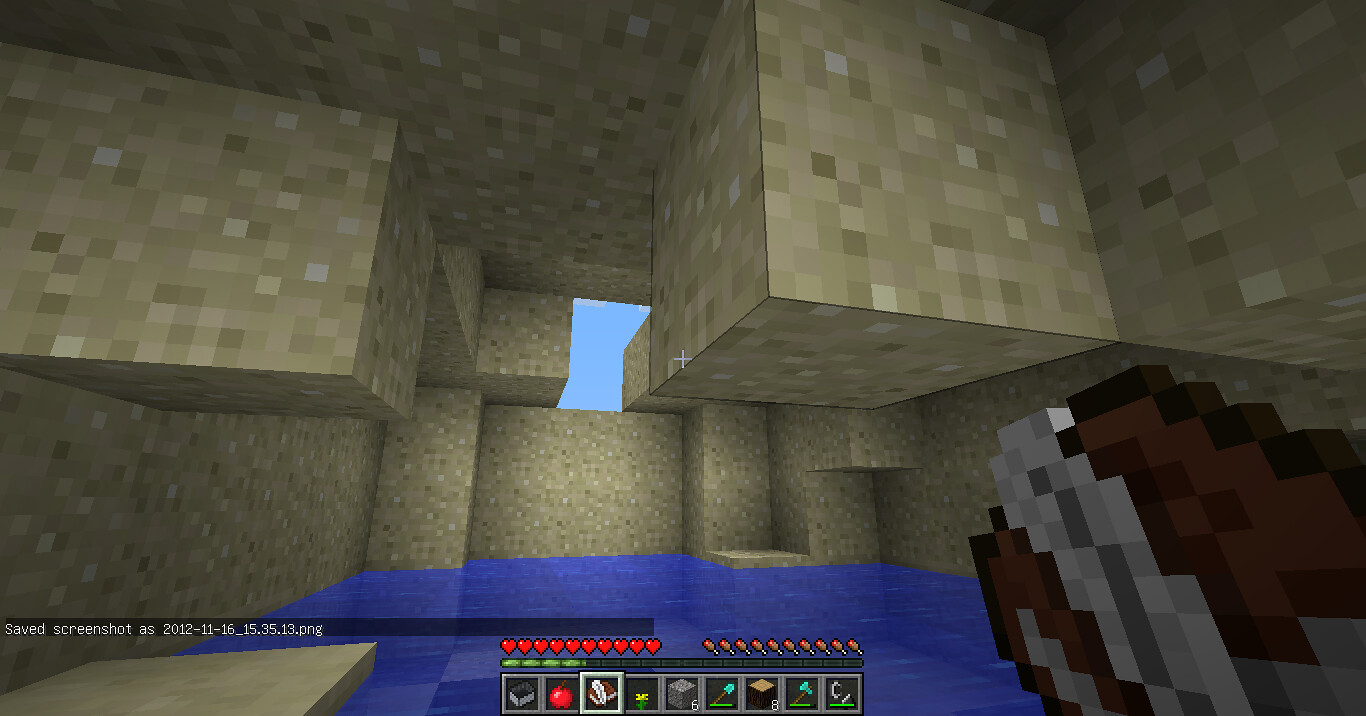This detailed screenshot from a video game depicts a complex scene featuring a large wall created from numerous small, square stones or tiles in shades of gray, light brown, beige, and light green. A distinct blue, hexagonal shape interrupts the pattern in the wall. The scene includes a pixelated stone walkway with many ridges and steps, leading towards a flooded area at the bottom of the image, indicating the presence of water. A health bar at the bottom shows multiple hearts, suggesting the character is healthy. Accompanying this bar are various symbols and icons, including what looks like an apple, a gray square box, and a yellow flower, though their exact functions are unclear. In the lower left, text reads, "Screenshot. Save screenshot as 2012 11 16_15.35.13.png." A blurry, maroon, and gray cartoon-like object is visible on the lower right, adding to the intricate, Minecraft-like design of this maze-like fort scene.